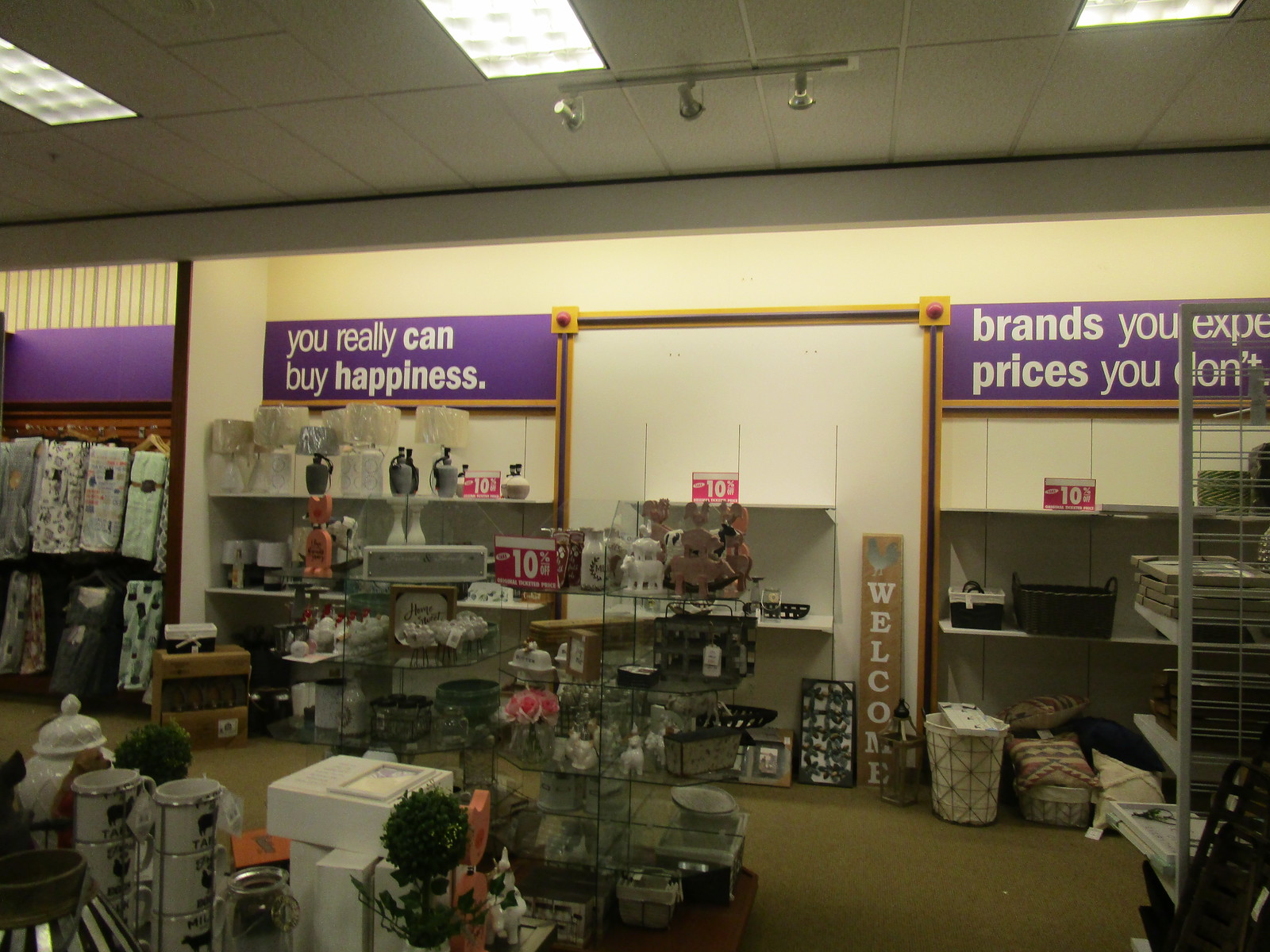This photo captures the bustling interior of a home goods and decor section of a store. The light brown floor is dotted with multiple stacks of merchandise, creating a crowded clearance area. Overhead, the ceiling features three vertical fluorescent lights providing ample illumination. The top middle of the far wall is adorned with three prominent purple rectangular signs, the first of which reads "You really can buy happiness" in white text, while another states "Brands you expect, prices you don't."

The wall beneath these signs is lined with an array of house goods. There are shelves holding lamps, baskets, and linens, along with various artworks and a vertical welcome sign that leans casually against the wall. This sign is light brown with the word "Welcome" written vertically in white. To the right, there are partial wire racks, and to the left, various towels are hanging.

In the foreground, on the left, there is a display of cups, vases, and glass containers. The right side of the wall further houses baskets and other home essentials. Scattered among the merchandise, small pink clearance signs announce a 10% discount, adding to the vivid and busy atmosphere of this well-stocked store section.